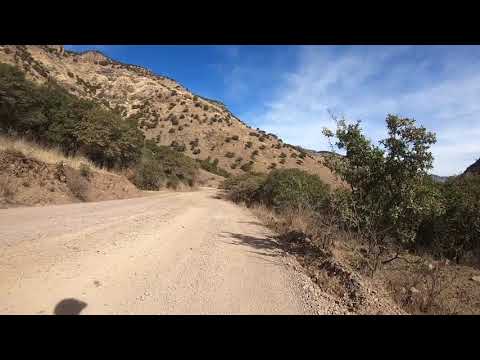This image captures a barren, sun-drenched landscape, possibly a hill or mountain, dominated by shades of beige, tan, and brown. A light sandy dirt road, grainy and seemingly seldom traveled, extends toward the center of the photo, flanked by sparse vegetation. On the left, undulating hills appear, their dry surfaces patched intermittently with brownish-green foliage, indicating a lack of vibrancy and aridity. The right side of the road features a mix of small green bushes and tiny trees, leading towards a slight drop-off. In the distance, a larger mountain looms, its surface dotted with scattered low bushes and grasses, all maintaining the same muted color palette. The sky above is a vivid blue, accented by a thin layer of wispy white clouds. Near the edge at the bottom of the image, the shadow of an unmistakable human head or a hat casts onto the road, hinting at the photographer's presence amidst this desolate yet picturesque scenery.